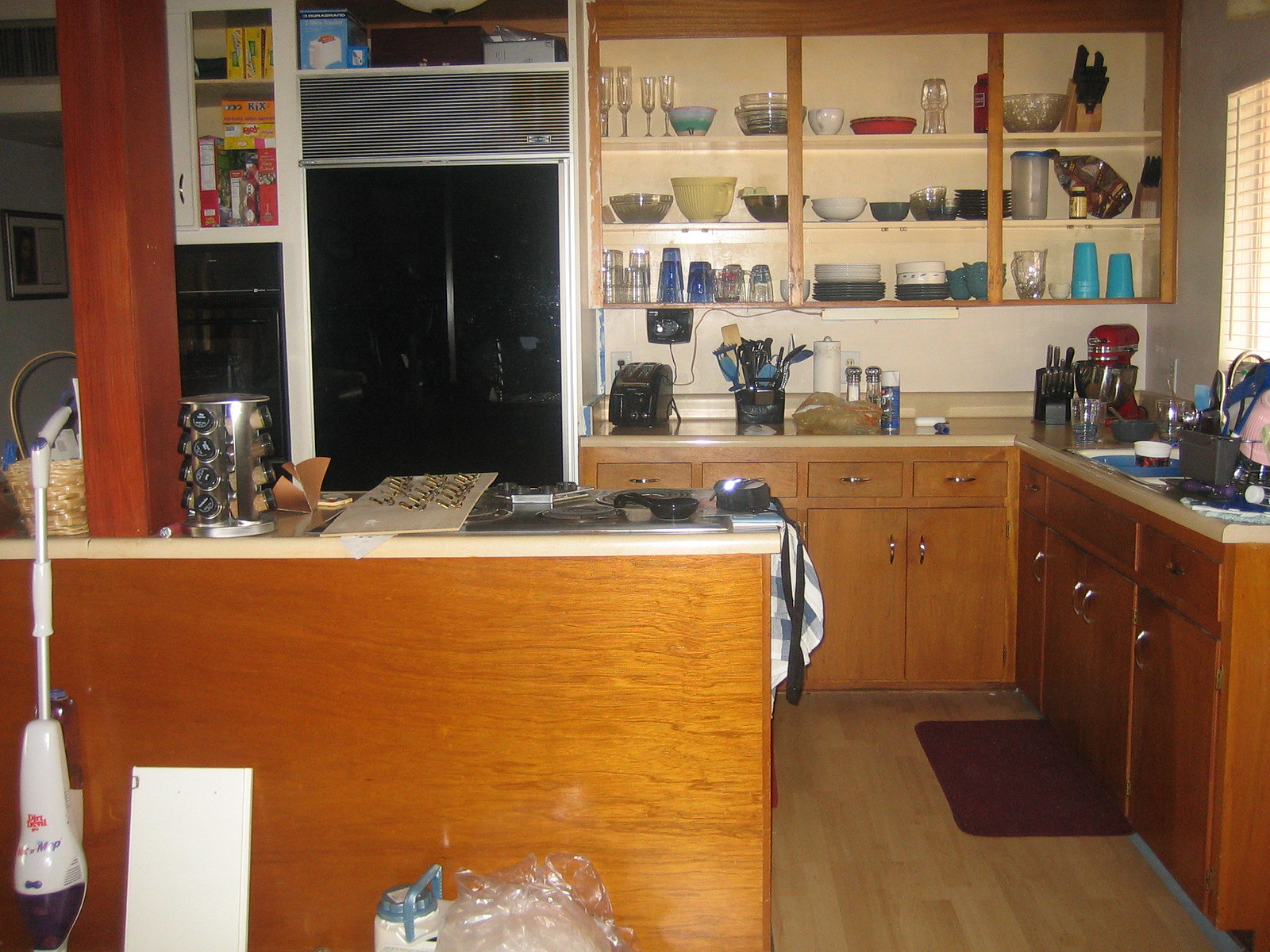The image depicts a well-organized kitchen, characterized by its wooden cabinets lining the back wall, arranged in three vertical sections, each with three open shelves.

In the left section:
- The top shelf houses four tall glasses, positioned next to several smaller bowls, followed by larger glass bowls.
- The middle shelf is occupied by a collection of bowls, including a large black glass bowl and a sizable yellow bowl with a handle, reminiscent of a large mug.
- On the bottom shelf, various glasses are stacked on top of each other.

In the center section:
- The top shelf features various glassware and several flat bowls, similar to pie dishes.
- The middle shelf contains a variety of bowls.
- The bottom shelf is lined with plates.

In the right section:
- The top shelf showcases a large bowl and a block of knives.
- The second shelf supports a pitcher, an additional block of knives, a package, and a bottle of vitamins.
- The bottom shelf contains a glass pitcher and multiple glass cups, neatly stacked.

Below the shelving units, lower cabinets are visible, along with a sink. A black refrigerator stands prominently in the center of the kitchen. An island, equipped with a stove, completes the scene, adding both functionality and a touch of modernity to the space.